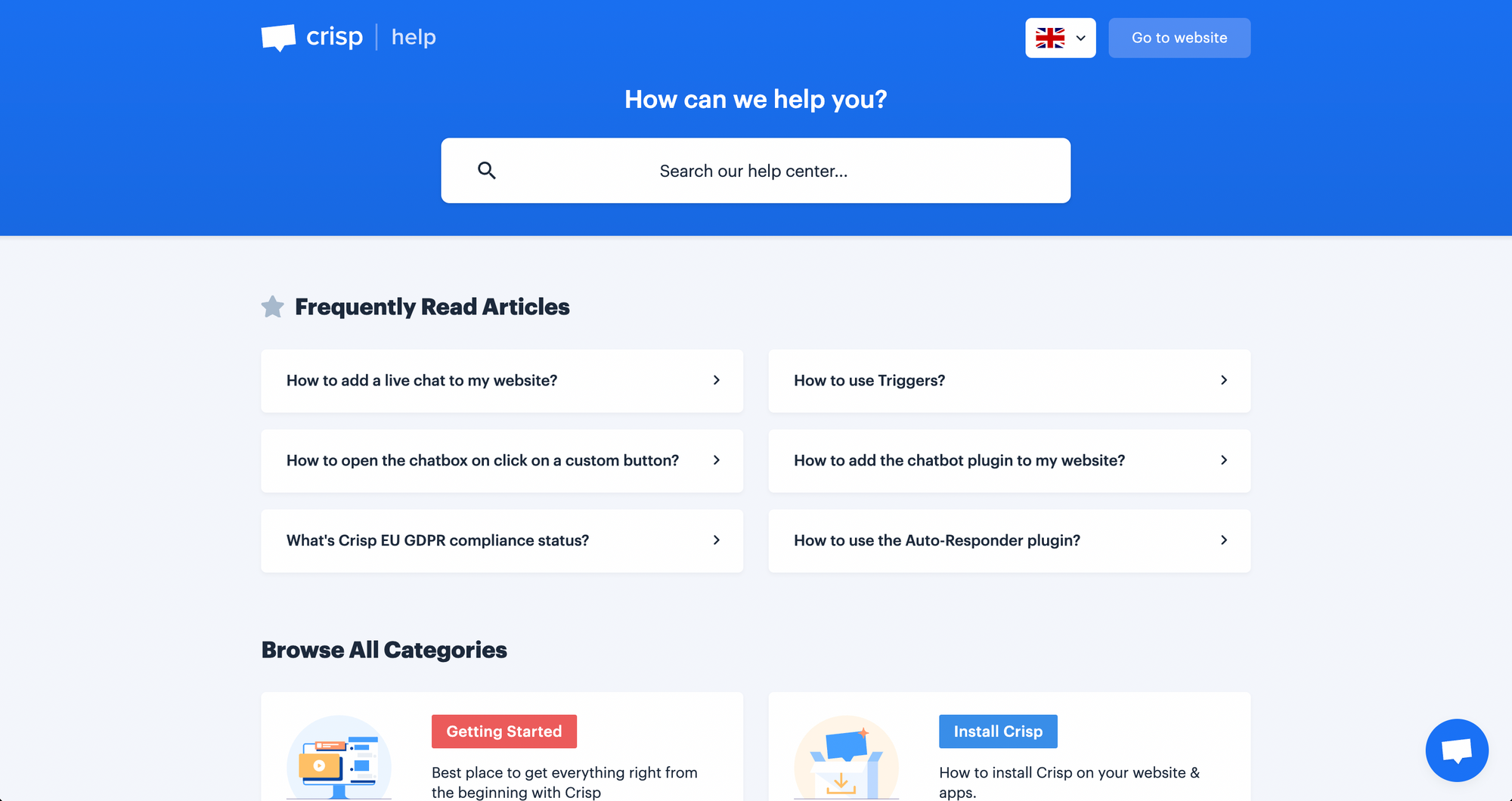This image is of a help website with a clear and structured layout. In the upper left corner, slightly shifted more towards the center, there is a logo that reads "Crisp" followed by a slash and the word "help." This logo and text are presented in white. Positioned centrally in the header, there is a text prompt that says "How can we help you?" in white, aligned with a large white search bar beneath it that reads "Search our help center."

In the upper right section above the search bar, there's a dropdown featuring the UK flag and to its right, a button that says "Go to website" in white text. Below the header, the main body of the page has a white background and begins with a bold title stating "Frequently Read Articles." Below this header, six articles are displayed in two columns, with three items in each column. Examples include "How to add a live chat to my website" in the left column, and "How to use triggers" in the right column.

Next, the section titled "Browse All Categories" is in bold black text, under which two categories are listed: "Getting Started" and "Install Crisp." In the bottom right corner of the page, there is a circular icon with a blue background and white text.

The overall design is clean, with a centered layout and regular use of white text against a darker background for headers and navigational elements.